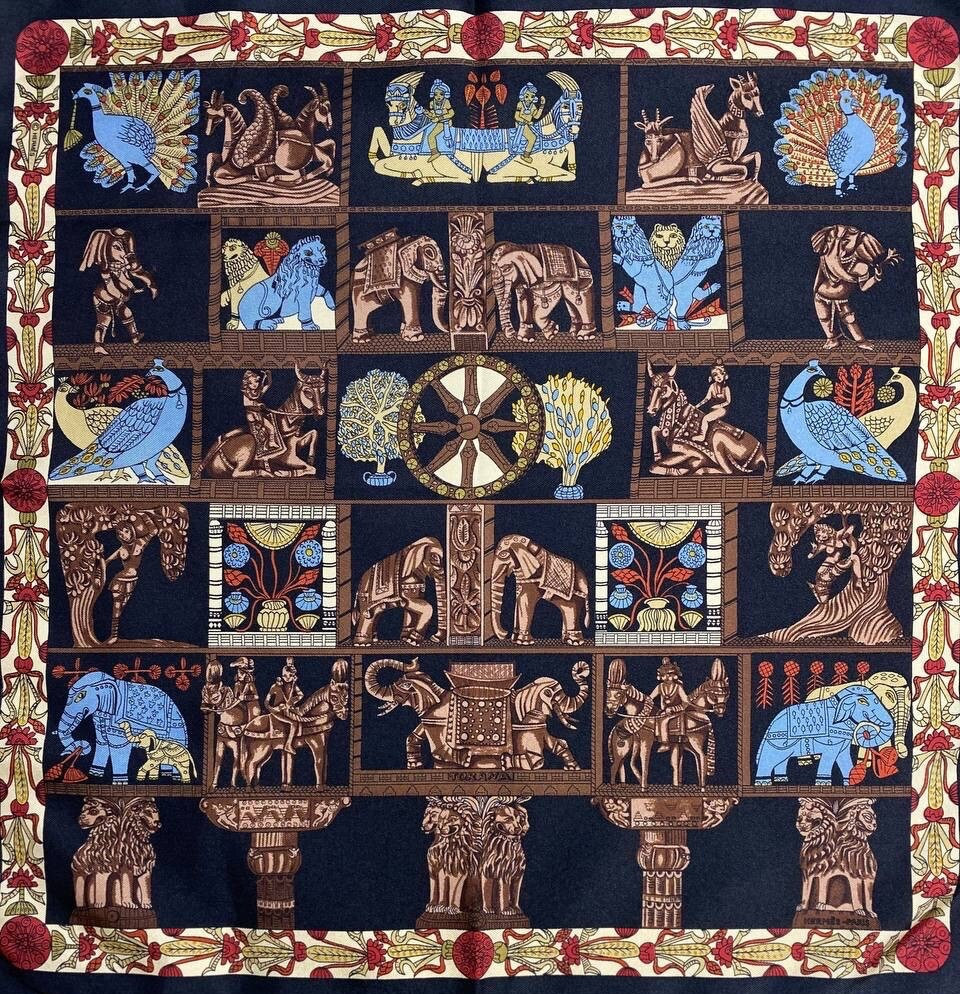This image depicts what appears to be an artistic tapestry or possibly a book cover, characterized by a rich and intricate design. The tapestry features a border with beige and mauve colored patterns, accented by mauve circles positioned at the corners and quarters (12, 3, 6, and 9 o'clock positions). Inside the border, the main background is a deep, navy blue, almost black. The central design is composed of numerous decorated squares and rectangles, each containing various artistic illustrations.

The decorations inside these sections predominantly showcase motifs in bronze, light blue, light beige, and tan hues, with additional accents in red and yellow. The illustrations include a variety of animals like peacocks, elephants, goats, and possibly lions, as well as a man and a mythical creature with three heads. The designs appear drawn rather than photographed, contributing to an overall detailed and complex visual narrative. 

One notable feature is a strip along the bottom of the tapestry that contains four distinct designs, which suggest an Asian influence. The artwork's organization, with varied square and rectangular sections, lends it a resemblance to a calendar or a book cover, particularly since there's a visible crease in the middle hinting at the folded layout of a book. Overall, the intricate detailing and diverse array of motifs make it a captivating and visually rich piece.